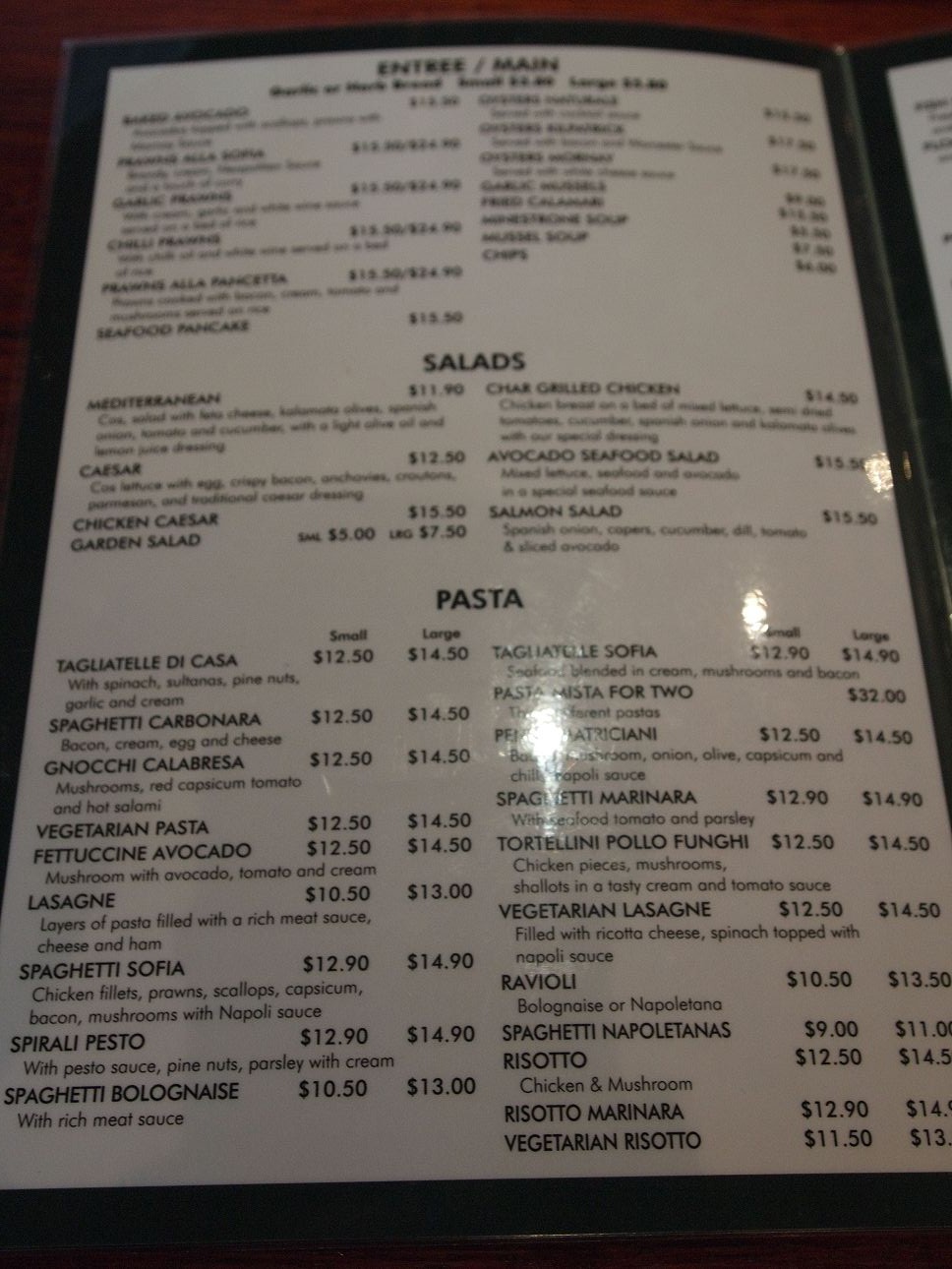This captivating image showcases one side of a restaurant menu, elegantly displayed on a dark brown table that peeks through as a border near the top and left side. The menu is rectangular, framed with a sleek black border and featuring a clean white background. The text is printed in bold black, offering a clear contrast for easy readability.

At the top, despite some blurriness, the section labeled "Entree Main" is faintly visible. The specifics of the dishes in this section unfortunately cannot be discerned due to the blurriness.

Moving to the next section, "Salads," a variety of fresh options are listed with their respective prices:
- Mediterranean Salad: $11.90
- Caesar Salad: $12.50
- Chicken Caesar Salad: $15.50
- Garden Salad: Small - $5.00, Large - $7.50
- Char-Grilled Chicken Salad: $14.50
- Avocado Seafood Salad: $15.50
- Salmon Salad: $15.50

Following the salads, the "Pasta" section offers a delicious assortment of pasta dishes, each available in small and large sizes. The dishes featured include:
- Tagliatelle di Casa
- Spaghetti Carbonara
- Nocci Calabresa
- Vegetarian Pasta
- Fettuccine Avocado
- Lasagna
- Spaghetti Sofia
- Spirali Pesto
- Spaghetti Bolognese
- Tagliatelle Sofia
- Pasta Mista: $2.00
- Spaghetti Marinara
- Tortellini Pollo Funghi
- Vegetarian Lasagna
- Ravioli
- Spaghetti Napolitana 
- Risotto
-- Chicken and Mushroom
-- Marinara
-- Vegetarian

This meticulously detailed menu entices diners with a range of salad and pasta selections, ensuring that every palate finds satisfaction among these savory offerings.